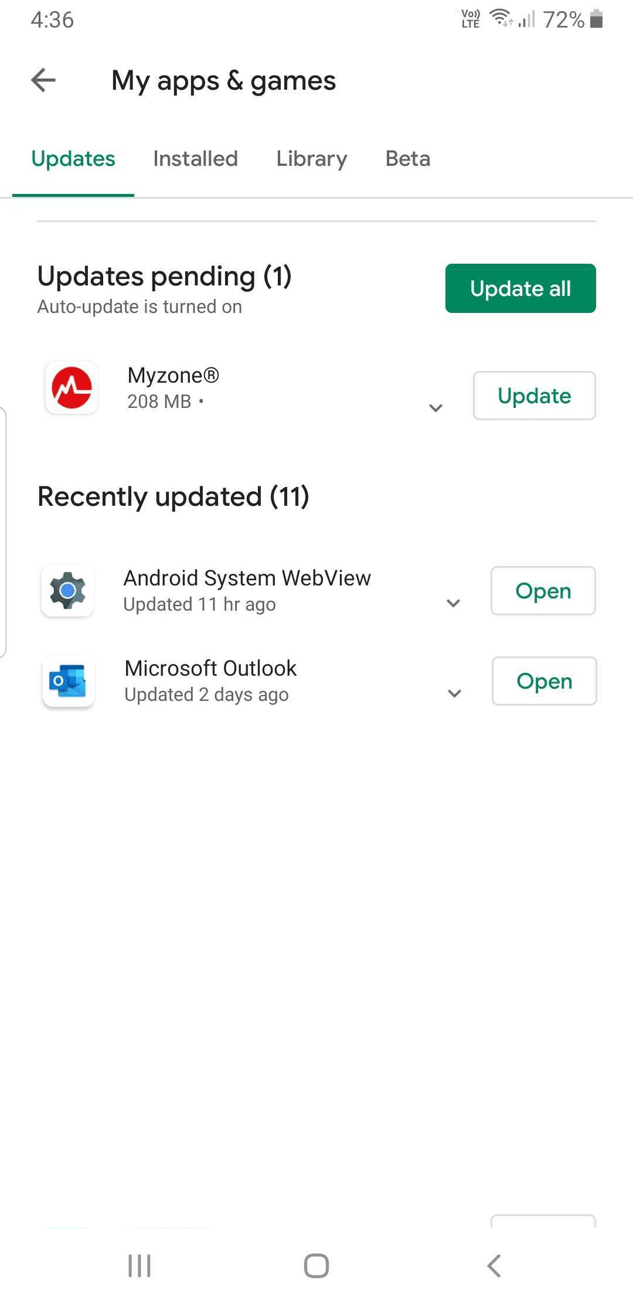The image showcases a user interface screen displaying various system updates and app management options. In the upper left corner, the time is displayed as 4:36, while on the right, the battery level is at 72%. Below, there is a leftward-facing arrow next to the text "My Games & Apps" written in black. 

Beneath this title, there's a green section labeled "Updates" with both the text and the underline in green. To the right of this section, there are the words "Installed," "Library," and "Beta." Below this header, in black text, is "Updates Pending" with the number "(1)" beside it, indicating a single pending update. The option for Auto-update is turned on, and a prominent green rectangle contains the white text "Update All."

Additionally, there's a red circle with a line through it labeled "My Zone," showing 208 MB of data, alongside an option to update. Further down, a section titled "Recently Updated" indicates "(11)" updates in parentheses. 

Among the updates, there is an image of a circle resembling a wheel, representing "Android System WebView," which was updated 11 hours ago. To the right of this entry is the option to open it. Next, "Microsoft Outlook," which was updated two days ago, also has an option to open it. The word "Open" is highlighted in green text in both instances.